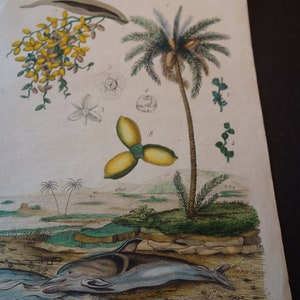The image is a detailed, hand-drawn sketch on white paper, depicting a beach scene. At the bottom left, a gray dolphin with a blue belly is beached on yellowish-tan sand, facing left, with a small sliver of water beside it. A tall palm tree with a brown trunk and lush green fronds stands prominently towards the right, rooted in a circular patch of green grass. In the middle of the image, a flower with three yellow pinwheel-shaped petals and a green center adds a focal point. The background features several small penciled-in palm trees and patches of greenery atop the tan ground. Additionally, the top left corner of the image showcases some yellow flowers on green vines, and a few yellow blossoms appear to float freely in the sky, contributing to the whimsical nature of the scene.